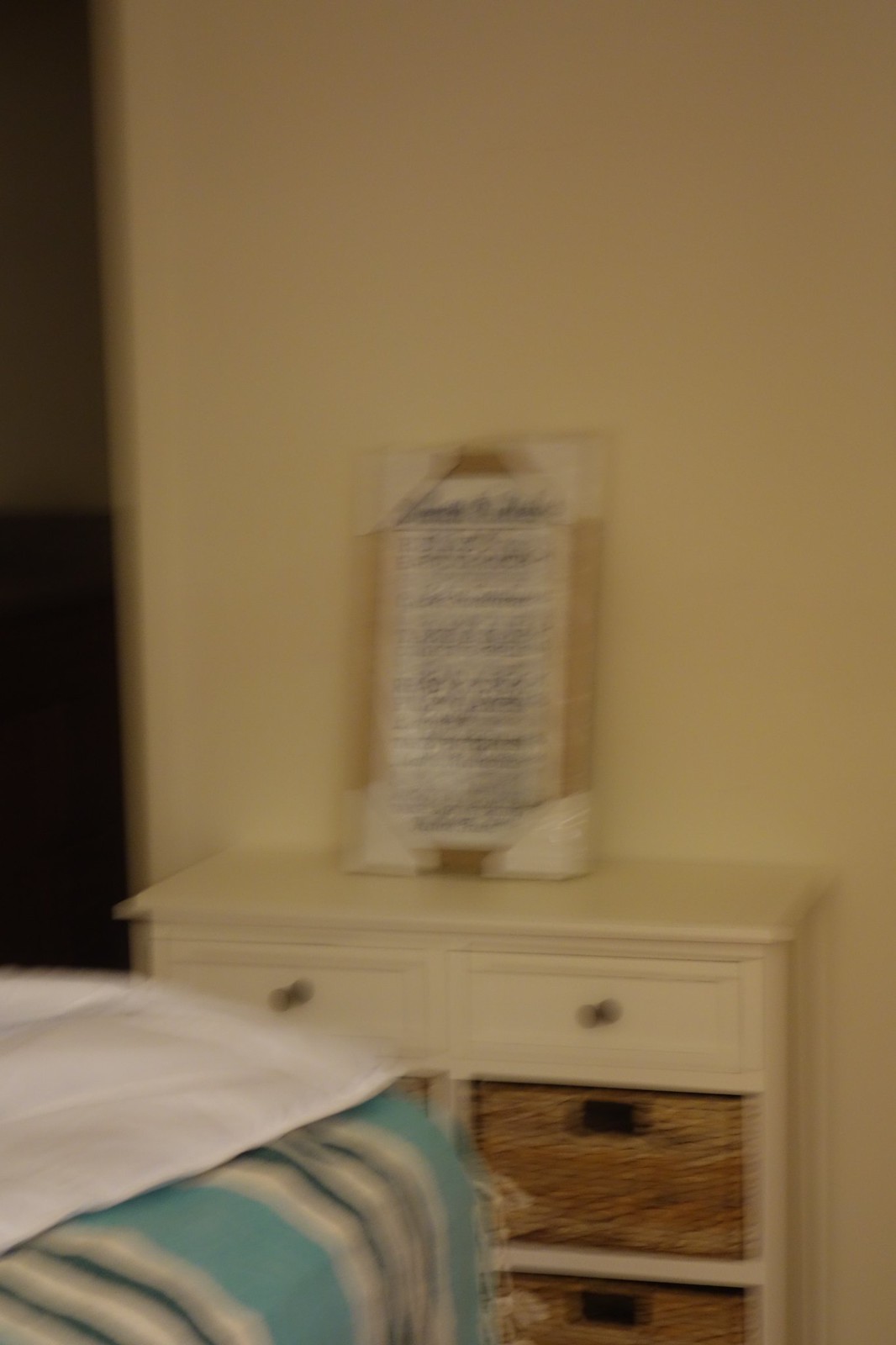The image is a color photograph taken indoors, oriented in portrait format, and notably out of focus, giving the setting a blurred appearance. The scene is likely set in a bedroom, discernible from the furniture and elements visible. Central in the image stands a white chest of drawers that features two pull-out drawers at the top and cubby holes below, each occupied by tan wicker basket crates. These crates showcase handle cutouts in shadow, indicating ease of removal. The chest has two columns of these cubby holes; the right column extends out of the frame while the left is partially obscured by what appears to be the edge of a bed, draped partially in a striped bedspread. The bedspread sports alternating stripes of white, dark green, teal, and blue, over a white sheet.

Leaning against the wall on top of the chest of drawers is a framed piece of artwork, seemingly protected with cardboard corner guards, suggesting it has recently been purchased. This artwork has a white background featuring text in various handwritten styles, although the blurriness prevents the text from being legible. The wall behind the furniture is a yellowish-brown color, contributing to the cozy, warm feeling typical of a bedroom setting.